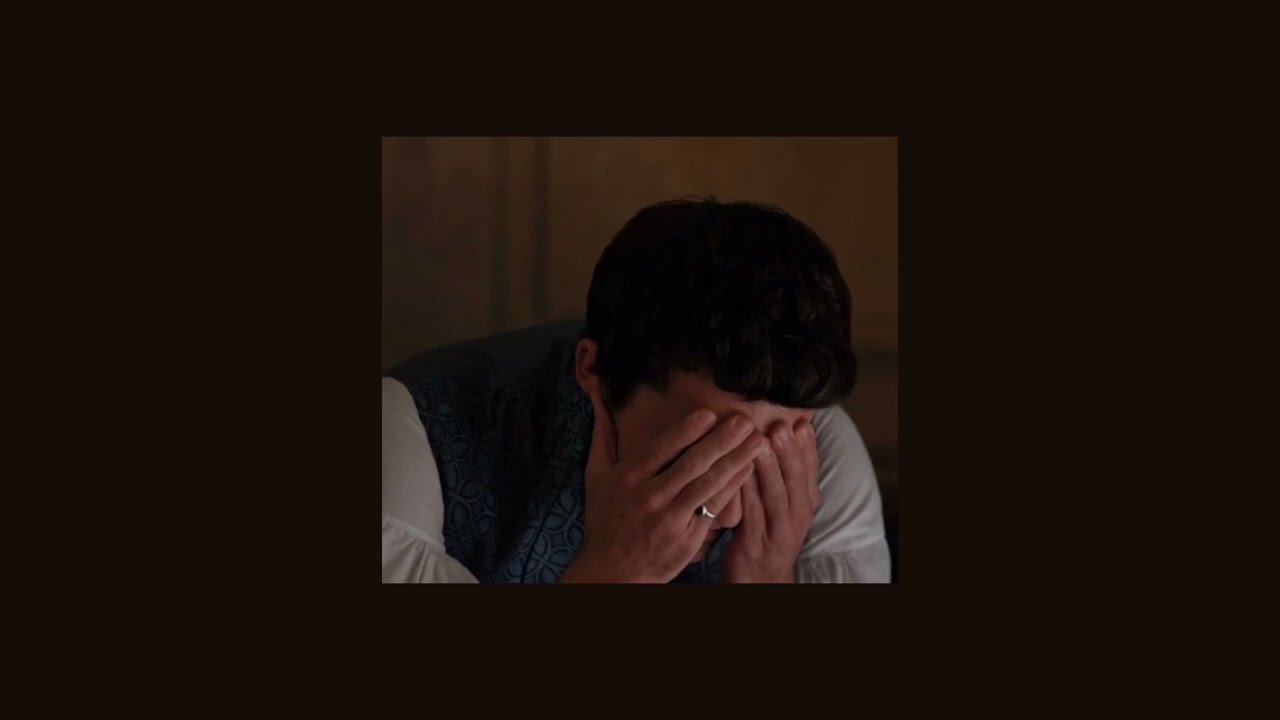In the center of a dimly lit, heavily letterboxed image, a young man is depicted in a state of apparent distress. Leaning forward with his head in his hands, his face is almost completely obscured, save for a small glimpse of his nose peeking through his fingers. His hands, covering his eyes, suggest he might be crying or deeply sad. He sports a gold ring on the pinky finger of his right hand. The man has short black hair and wears a white button-down shirt with puffy sleeves beneath a blue-green vest that could be reminiscent of 1800s period attire. The backdrop features a dark brown wooden wall with visible slats, enhancing the somber mood of the scene. His posture and the detail of his attire add to the evocative nature of the image, conveying a poignant moment of sorrow.